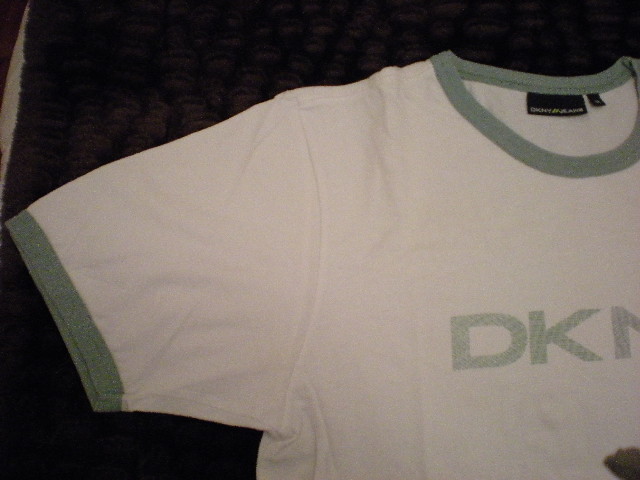This image features the upper portion of a slightly wrinkled, short-sleeved white t-shirt, positioned against a dark, textured background, possibly a black rug, brown towel, or bath mat. The t-shirt has gray or teal green borders on the sleeves and crew neck. Across the chest in matching gray or green gingham-style letters, it reads "DKNY," though only part of the lettering is fully visible. There is also a black tag with white writing on it, affixed to the shirt. The overall scene is slightly blurry and a bit dark, adding to the textured appearance of the surfaces surrounding the t-shirt.